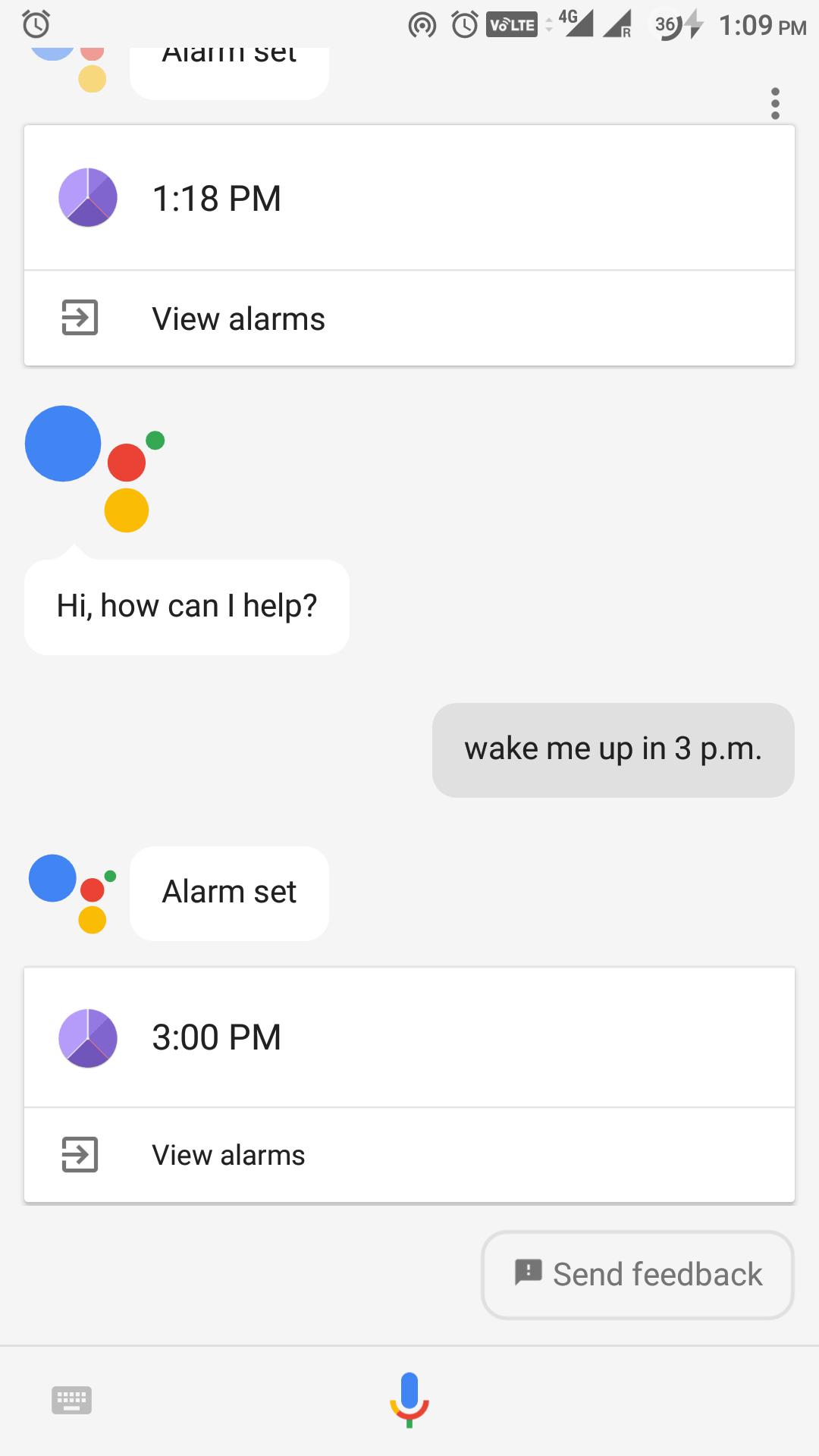The image depicts a simulated text exchange between a user and an AI assistant reminiscent of Google Assistant. At the top of the interface, there's a timestamp reading "1:18 PM." Below this, there's an icon labeled "View Alarms." On the left side, there are four small circles in Google's signature colors: blue, red, yellow, and green, indicating the AI assistant's presence. The assistant's text box is shown with the greeting, "Hi, how can I help?"

On the right side, the user's response appears in a gray text box stating, "Wake me up at 3 PM." The assistant then replies from the left again, confirming the action with "Alarm set." Directly beneath this confirmation is another box displaying "3 PM" followed by the text "View Alarms," indicating that the alarm has been scheduled successfully.